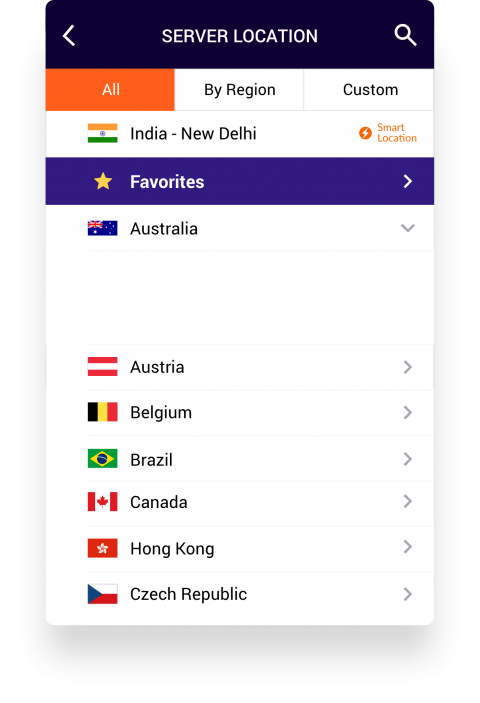**Detailed Caption:**

This image is a screenshot of a smartphone interface showcasing a server location selection menu. At the top of the screen, there is a navy blue header that features a left-pointing arrow, followed by the text "Server Location" in white, and a search icon positioned on the right side. Directly below this, an orange tab labeled "All" is prominently displayed, indicating the selected filter.

The main content area contrasts against a white background, with a few exceptions highlighted for emphasis. The first notable section is titled "Bi-Region Custom" and is marked with an orange box. Next, there is a smaller, navy blue box featuring a circular orange icon with a white thunderbolt on the right, next to the text "Smart Location." Below this is another navy blue box with a yellow star icon and the label "Favorites," accompanied by a right-pointing arrow.

The subsequent part of the list, still on a white background, consists of server locations for various countries. Each country has its flag icon before the country name. The list includes:
- India (New Delhi)
- Australia (with downward arrows)
- Austria
- Belgium
- Brazil
- Canada
- Hong Kong
- Czech Republic 

Overall, the interface is clean and categorized, with each section distinctly marked by different colored boxes and icons for ease of navigation.